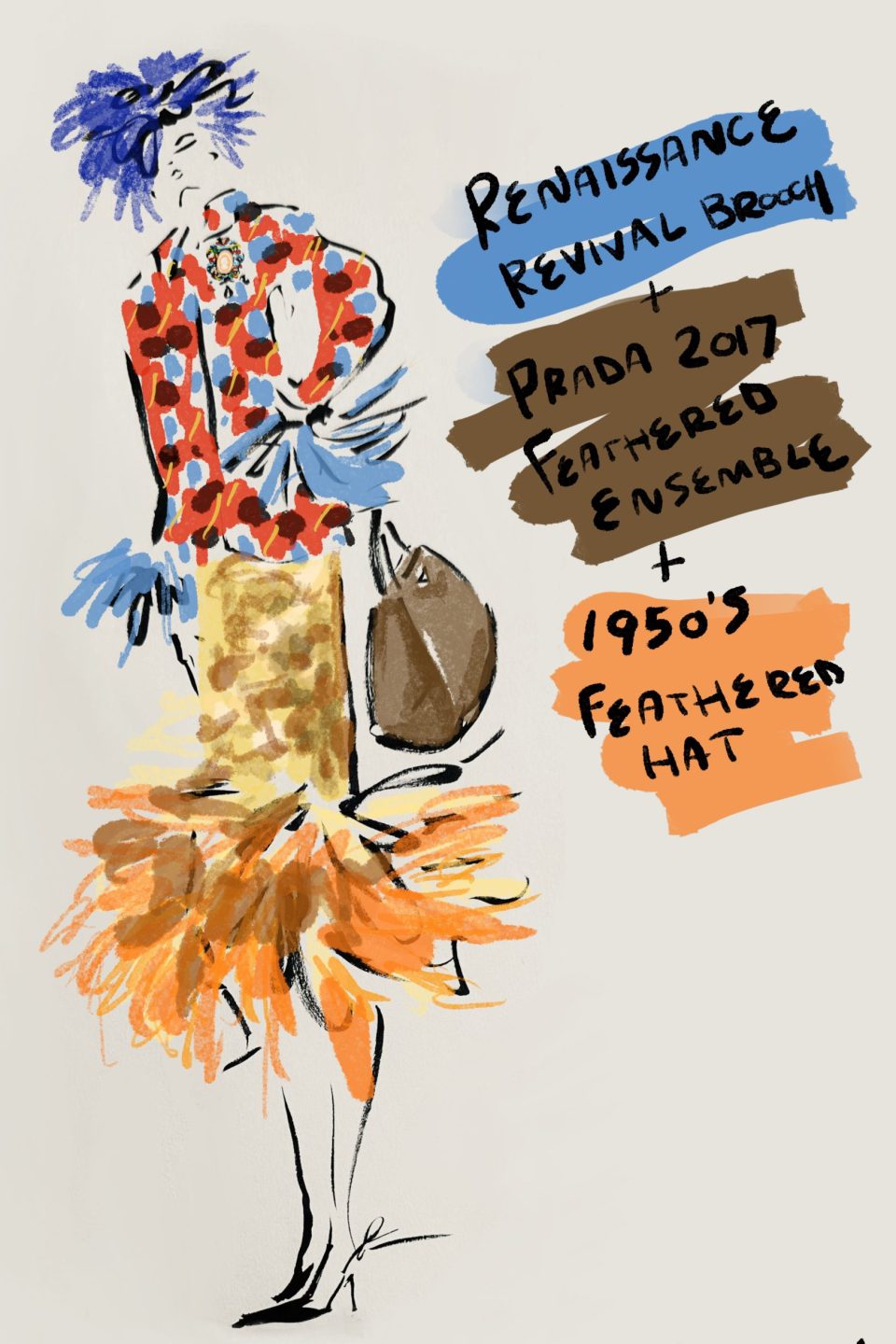The image portrays a very abstract, watercolor-style artwork of a woman with striking blue, wild hair that extends outward like a series of sparks. Her face, outlined in black with minimal details, suggests a neutral or slightly sad expression, enhanced by simple line strokes for facial features and the chin. She is attired in a colorful and eclectic ensemble, featuring a coat with red, blue, and brown spots, accented with poofy blue sleeves. Her outfit includes a tight skirt in white, yellow, and brown hues that flares out into a fluffy orange feather-like design at the bottom. She accessorizes with a brown purse tucked under her left arm and black high-heeled shoes. 

In the upper right corner of the image, set against a backdrop subtly painted in blue, brown, peach, and possibly lavender, there is notable painted black text. The writing, layered over streaks of various colors, reads "Renaissance Survival Roach," "Prada 2017 Feathered Ensemble," and "1950s Feather Hat." Despite variations, the core elements emphasize the piece's playful yet sophisticated blend of fashion and abstract art, capturing a whimsical, surreal aesthetic.